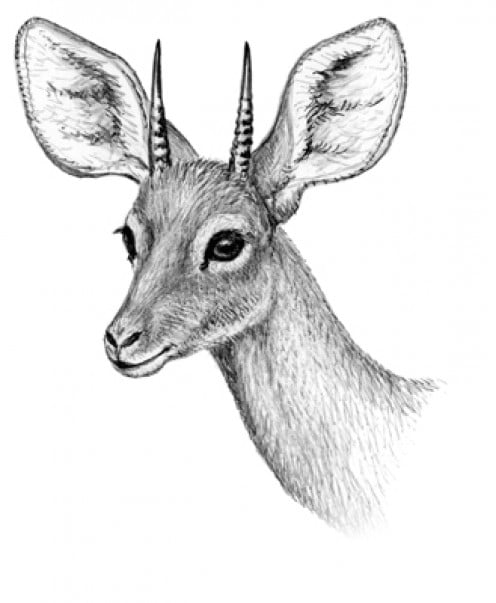This is a detailed pencil drawing of a deer head set against a solid white background. The composition is predominantly black and white, giving it a classic and striking appeal. The deer's large, almost bunny-like ears project upwards towards the upper left and right corners of the image. Between the ears, two small, grooved antlers extend slightly above the ear tips. The texture and shading create a three-dimensional effect, with dark sketches accentuating the inner parts of the ears.

The deer's head is tilted slightly, gazing towards the left, revealing its large, reflective left eye entirely and a portion of its right eye. The eyes stand out with dark irises and light rings around them. The closed mouth forms a slight smile without showing any teeth. The nostrils and the mouth are distinctly darker, lending more depth to the facial features.

The neck extends down towards the lower right corner but is cut off before the body begins, showing only the short, textured fur with subtle shading in brown and white patches. The overall sketch showcases intricate detailing, capturing the deer's serene yet expressive demeanor.